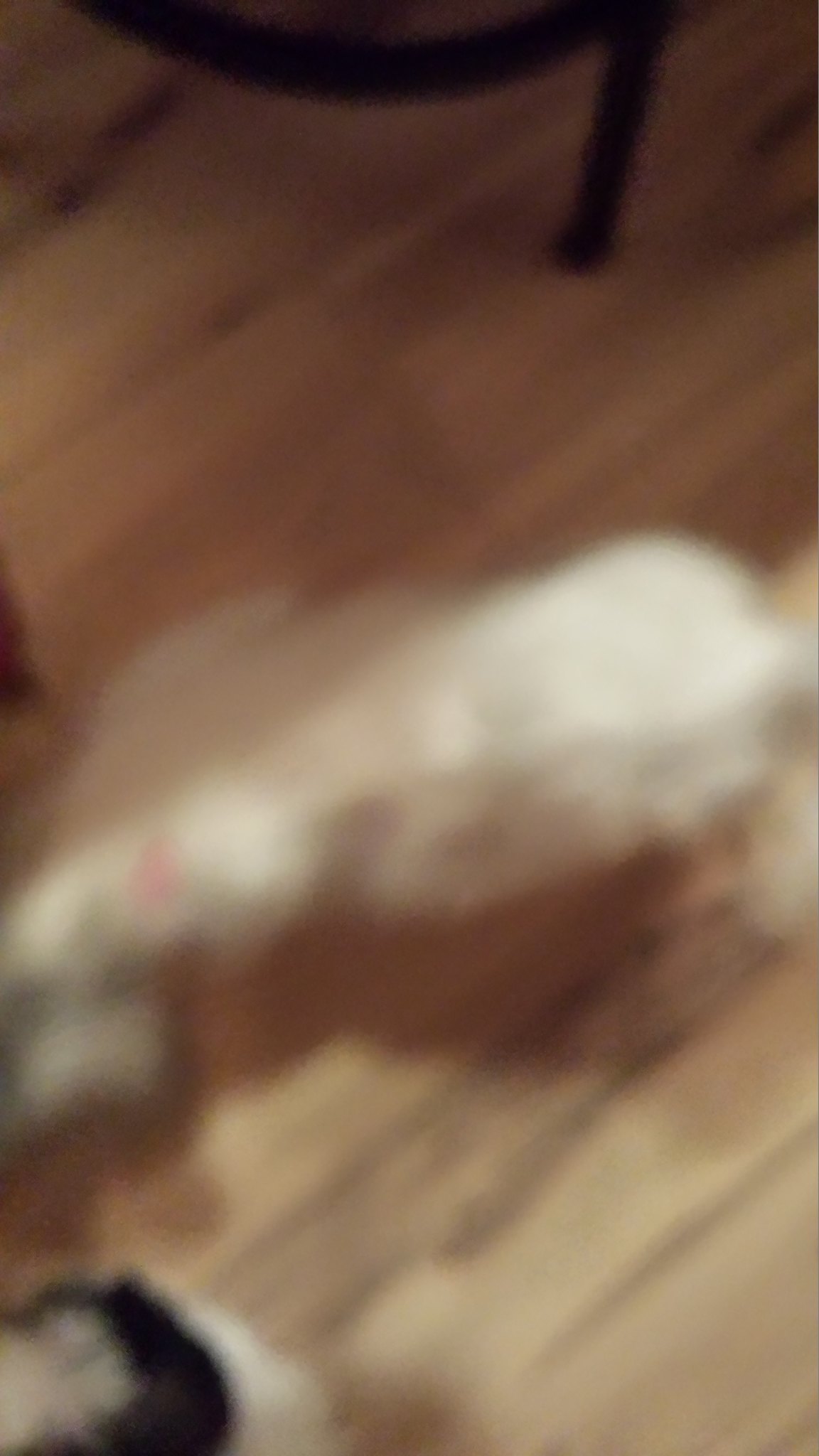This photograph depicts an out-of-focus, overhead view of a light cream-colored dog standing on a light whitish oak or possible simulated wood linoleum floor. The dog's head, which is slightly lower than its back end, is on the left side of the image, facing toward the right. The dog appears to have a pink or red bow on its head, although the blurriness makes it difficult to be certain. The flooring features dark streaks running through sections of it. In the bottom left corner of the photo, there is a black square with a beige center. At the top of the image, a black, half-circle leg of a chair or stand curves downward, adding a defined yet unclear element to the composition.